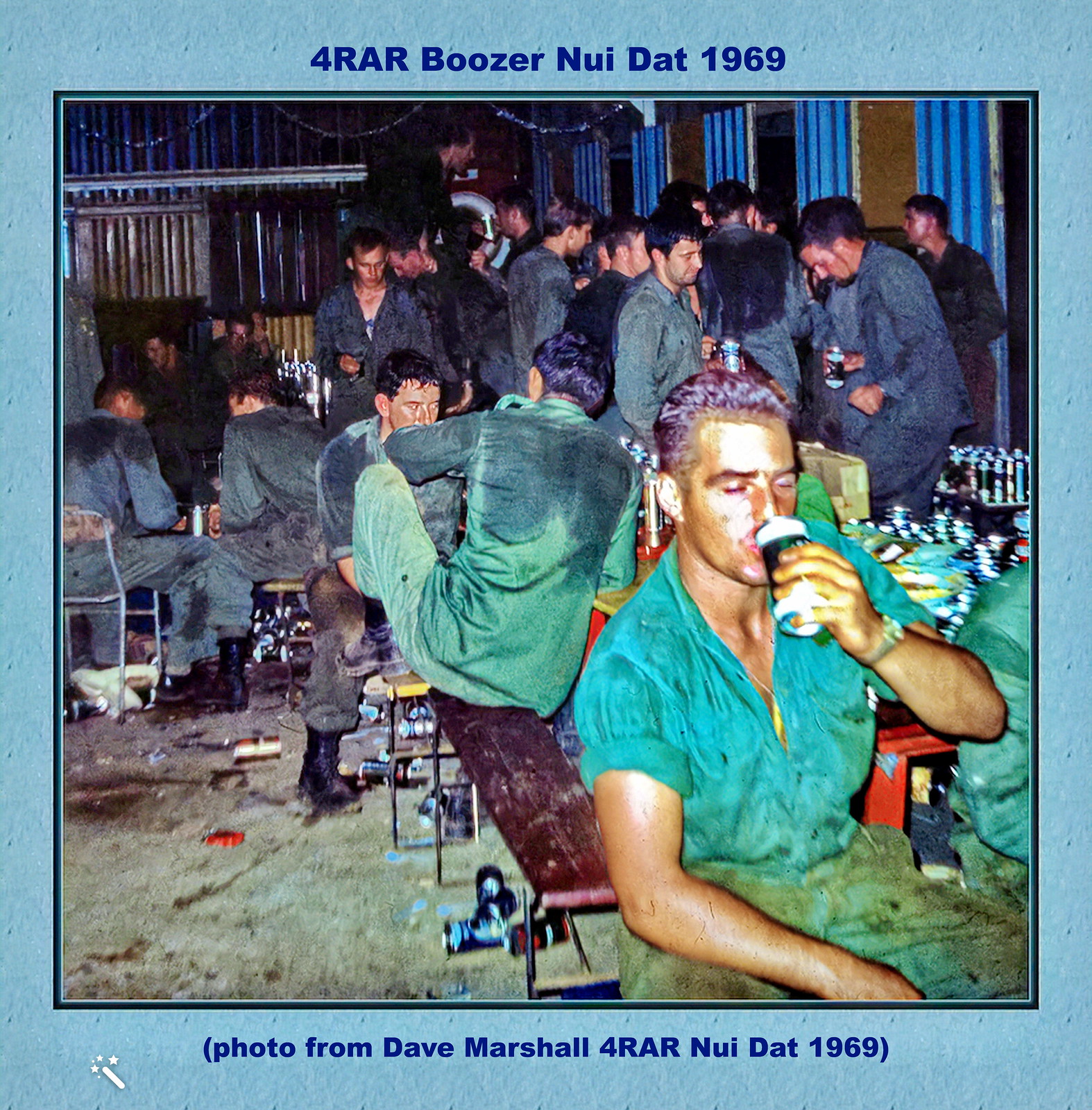The photograph, bordered in blue, captures a lively, crowded scene of what appears to be a makeshift bar or recreational area inside a tin shed. Men dressed in army uniforms with green shirts and pants are seen engaging in various activities. Some are drinking beer, and others seem to be playing games such as chess or checkers on the right side of the image. A prominent figure near the front, holding a beer with his sleeves rolled up to his shoulders, sports brownish hair and a wristwatch. In the background, clustered against the wall, is a group of men dressed in plain gray tops and bottoms, with many of their shirts stained or wet, possibly from sweat. The text embedded at the top of the photograph reads: "For R.A.R. Boozer, Newey Dat, 1969," while the bottom caption states: "(Photo from Dave Marshall. For R.A.R. Newey Dat, 1969)."